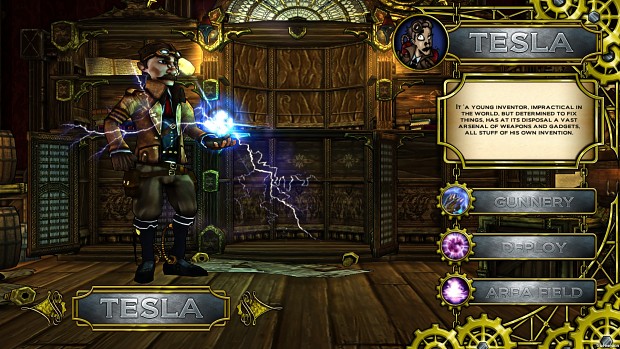This detailed screenshot from a video game features a character named Tesla, who is depicted as a mad scientist with a cartoony appearance. Tesla, a young inventor determined to fix things despite being impractical in the world, stands in his lair. He's attired in a brown jacket, gray pants, black boots, and has goggles on his forehead. He sports a mustache and holds a glowing bluish orb with lightning shooting out from his left hand, which appears on the right side from the viewer's perspective. 

The setting is a wooden-walled room with wooden floors, decorated with windows and carvings. On the left side of the image, there is a gray bar with a gold border that prominently displays Tesla's name in raised relief writing. Below this, Tesla's full body is visible, standing ready with his gadgets. On the right side, there’s another banner with Tesla’s name and a round inset showing his face. 

Underneath, a description reads: "A young inventor, impractical in the world but determined to fix things. He has at his disposal a vast arsenal of weapons and gadgets—all of his own invention." Below this caption are three labeled buttons: "Gunnery," "Deploy," and "Area Field," each decorated with gears contributing to the mechanical theme of the character and his environment.